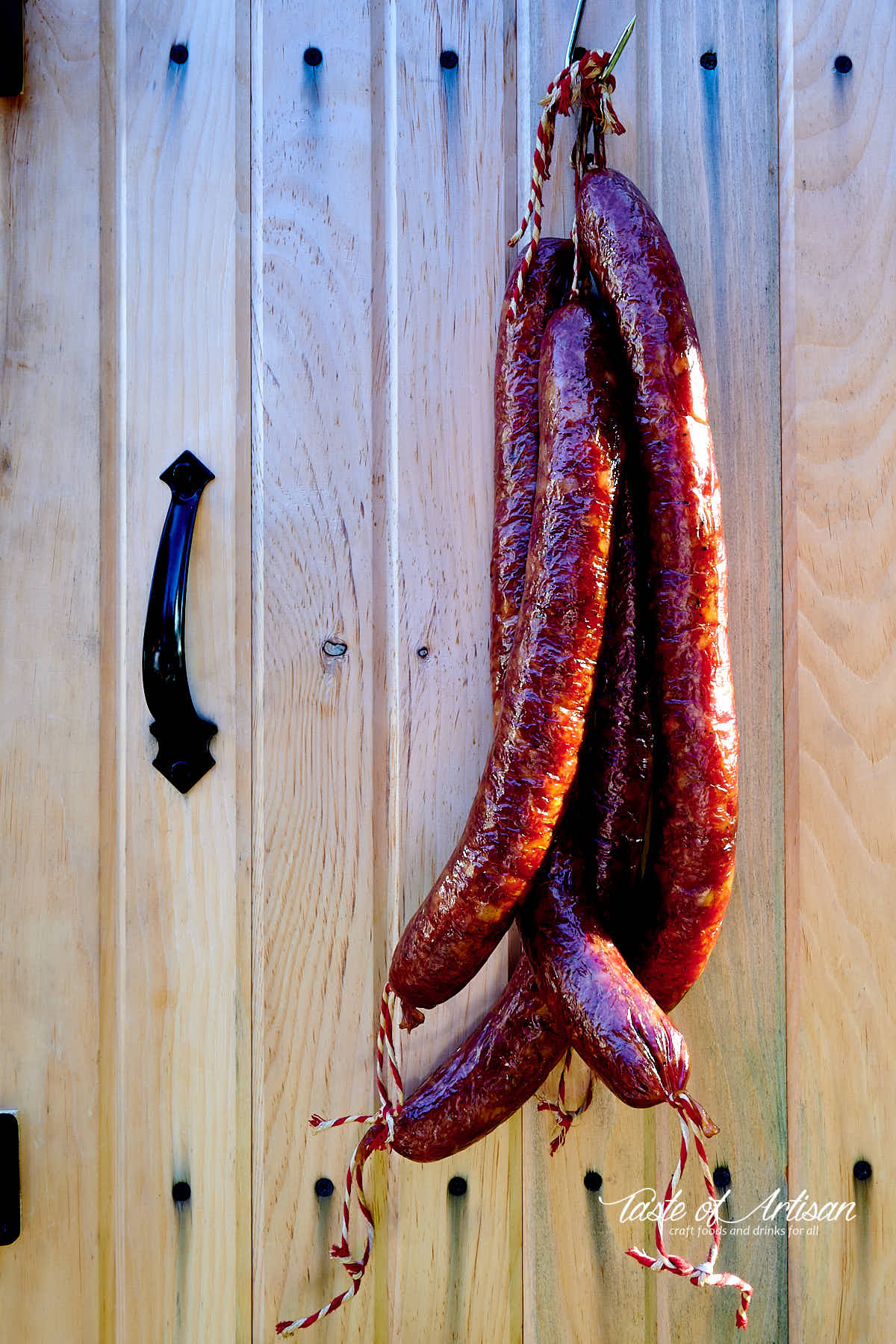This image features a close-up view of long, shiny sausages suspended from a sharp metal hook, resembling a large fish hook, in front of a light blonde wood-grain cupboard door with a high-polished black wrought iron handle at the bottom right corner. There are four sausages, encased in natural, glossy casings, each tied with striped red and white twine. The sausages, with a distinctive brownish-reddish-orange hue, dangle from a gold U-style hook at the top of the wood-paneled door, extending three to four times the length of the handle. The image evokes a sense of artisan craftsmanship, showcasing the rustic appeal and detailed presentation typical of traditional craft foods.